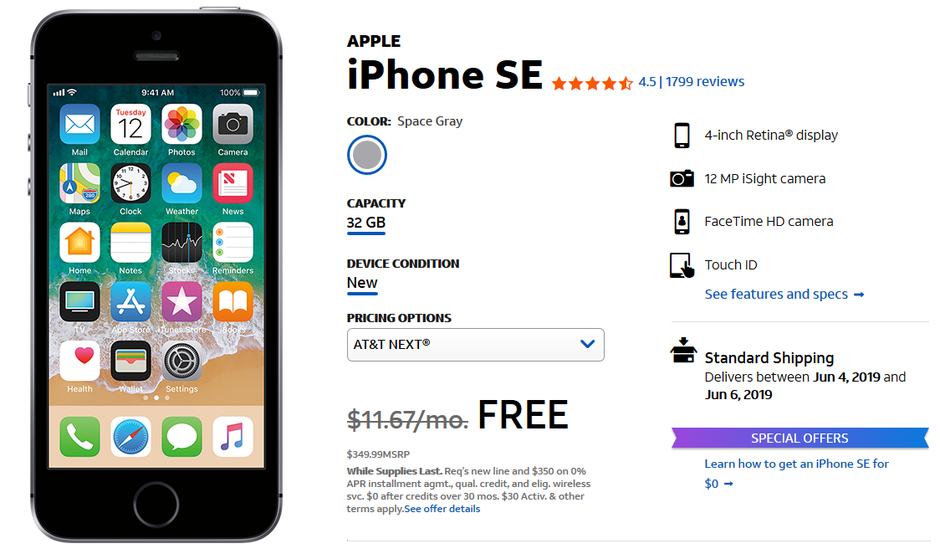The image features a horizontal rectangle with a white background. On the left side, there is an image of a cell phone with a screen densely populated with various app icons. To the right of the image, detailed product information for the Apple iPhone SE is displayed. The information includes:

- Model: Apple iPhone SE
- Rating: 4.5 stars 
- Number of Reviews: 1,799 
- Color: Space Gray 
- Capacity: 32 GB 
- Condition: New 

Pricing options are listed with an emphasis on a promotional offer:
- Original Monthly Cost: $11.67 (crossed out)
- Current Offer: Free 

Additionally, there's a mention of the full price (MSRP): $349.99 while supplies last, with specific terms and conditions including:
- Requires a new line and a $350 0% APR installment agreement.
- Qualifies with quality credit and eligible wireless service.
- The effective price is zero after credits over 30 months.
- Activation fee of $30 and other terms apply.

A blue link labeled "See offer details" appears for more information.

Highlighted features on the right side of the product details include:
- 4-inch Retina display 
- 12 MP Insight Camera
- FaceTime HD Camera
- Touch ID

A blue link labeled "See features and specs" with an arrow pointing right is also present.

Below this, there's a line followed by delivery information:
- Standard shipping delivers between June 4, 2019, and June 6, 2019.

Underneath, a note on special offers states:
- Learn how to get an iPhone SE for $0.